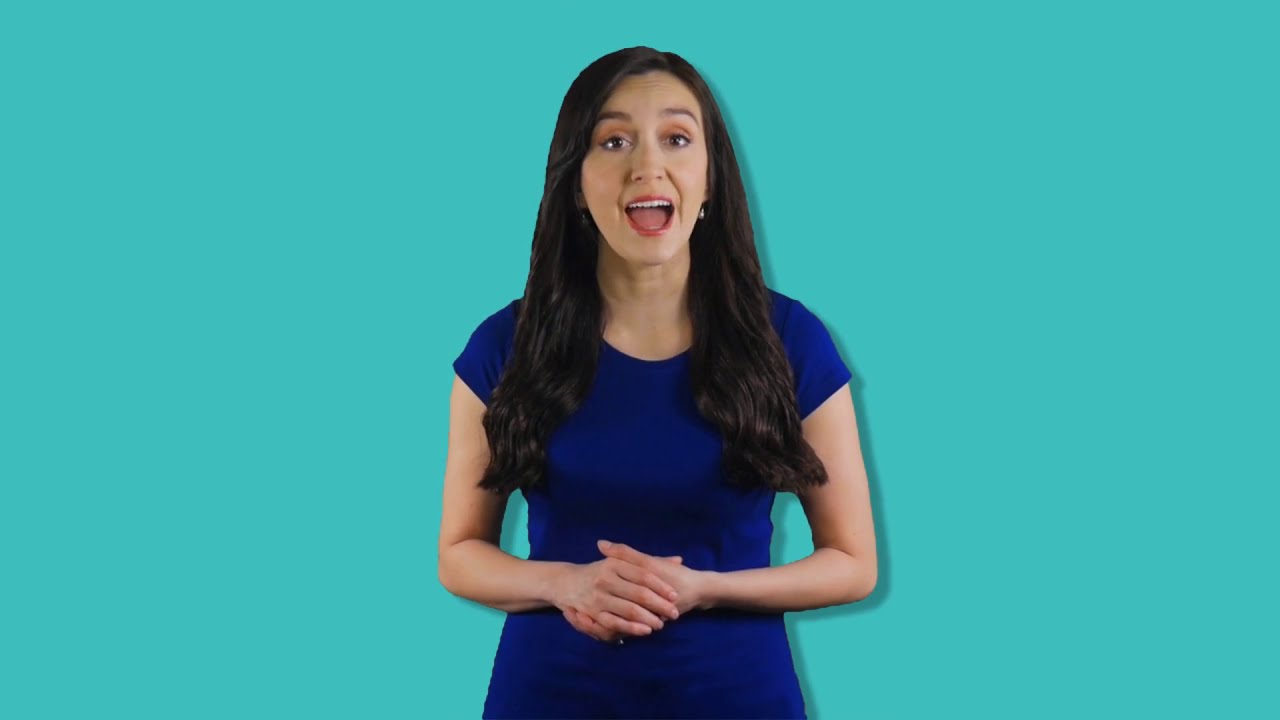The image captures a woman, most likely appearing in a still from a video, standing in the center of a horizontal rectangular frame with an all-turquoise or light teal background. The photograph is framed from her waist up. She has long, slightly wavy, brownish-black hair cascading down to her chest. Her mouth is wide open, revealing her white teeth and red lipstick, as if caught mid-speech. She has brown eyes highlighted with light brown eyeshadow, brown eyebrows, and small earrings in both ears. She is wearing a short-sleeved blue dress or t-shirt, with both elbows bent and hands clasped in front of her waist. The meticulous detail of her fair complexion and poised demeanor suggests a well-put-together individual, possibly conducting a tutorial or engaging in a video presentation.